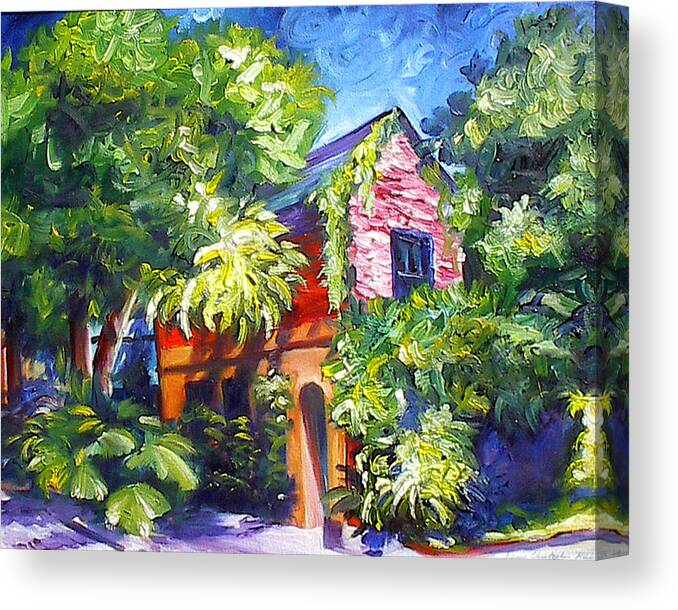This image depicts a vividly colored and textured canvas painting of a charming, two-story cottage set amidst a vibrant landscape. The house features a striking combination of colors: a pink front, a blue and purple roof, and red siding transitioning to brown at the lower level, which includes three openings. An archway, painted orange, adds an inviting touch to the entrance. The roof also has a blue and purple window. Surrounding the cottage, lush green trees with visible brown trunks, especially prominent on the left side, frame the scene. On the right, additional trees and green plants enhance the setting. The ground in front of the house is intriguingly depicted in purple, potentially suggesting either a road or water. Above, a blue sky with swirling white clouds completes the scene, further emphasizing the dynamic brushstrokes that characterize the painting. The edges of the canvas are squared off, giving it a three-dimensional appearance, and the artwork is noted for its swirly effect, reminiscent of brushstrokes. The painting itself stands out as a meticulously detailed, colorfully whimsical depiction of a house nestled in a natural, wooded area.